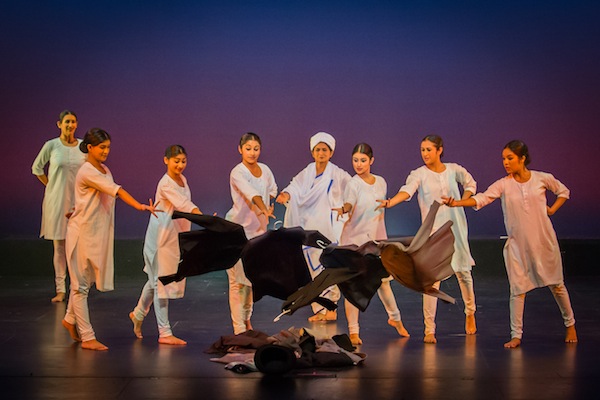A group of eight women are standing on a dark wood stage against a backdrop with a gradient from blue at the top to purple at the bottom. Seven of the women are dressed in long-sleeve white dresses paired with white pants, and they are in the process of tossing black jackets into a pile on the floor, using their right hands while their left hands are placed behind their backs. The woman in the middle stands out with a white dress that features blue borders, complemented by a white scarf and a hat. On the far left, slightly behind this line of women, another woman can be seen, dressed in a light green salwar kameez. The reflective stage floor amplifies the impact, mirroring the action and attire of the women. Additionally, pinkish lights add a dynamic visual accent to the scene.